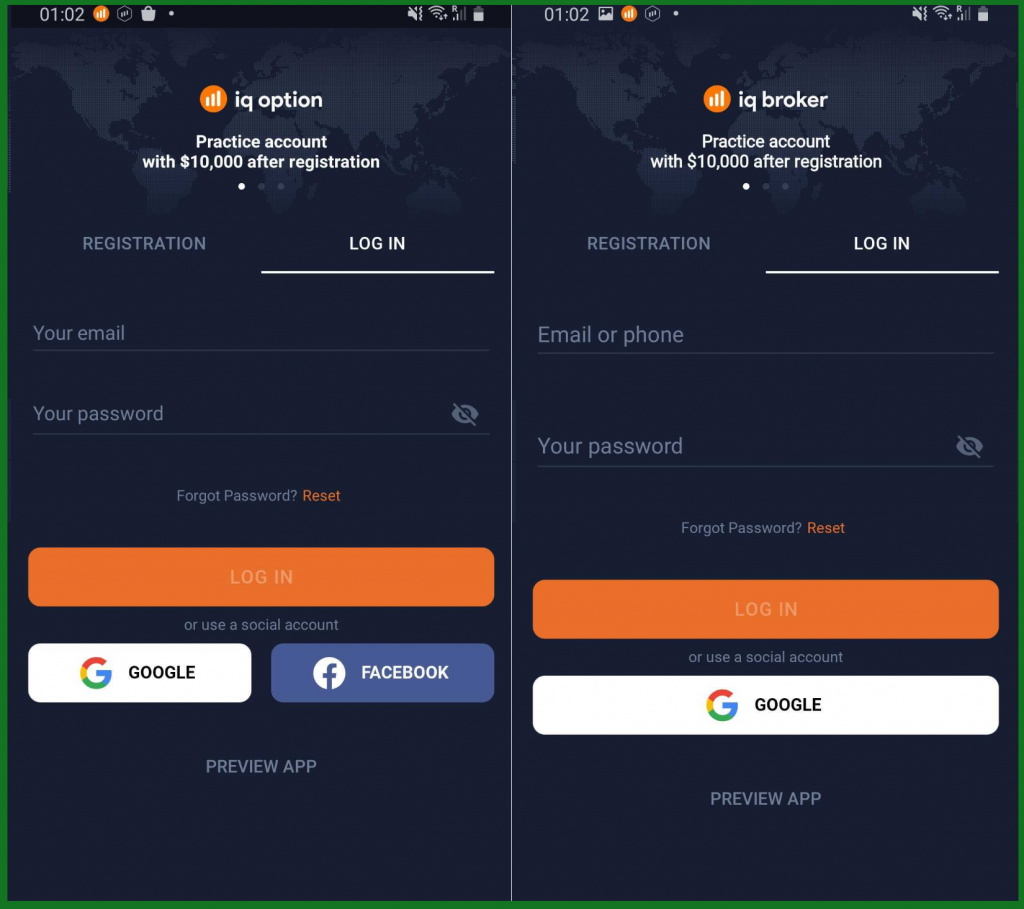The image consists of two screenshots, each displaying a login interface for an IQ Option practice account. Both screenshots show a time of 10:02.

**Screenshot 1:**
- Background: Light theme.
- Header: "IQ Option - Practice Account"
- Account Info: Indicates a balance of $10,000 for practice after registration.
- Navigation Dots: One white dot followed by two gray dots, signifying the user is on the first screen of a carousel.
- Sections:
  - "Registration" and "Login" options. The "Login" option is highlighted in white.
  - Input Fields: "Your email" and "Your password."
  - Links: "Forgot password?" which leads to a "Reset" option highlighted in orange.
- Buttons: 
  - "Login" button in an orange rectangle.
  - Option to use a social account for login, with buttons for "Google" and "Facebook" each in a respective rectangle.
- Footer: "Preview App."

**Screenshot 2:**
- Background: Dark blue theme.
- The layout and elements closely resemble those of the first screenshot.
- Deviations: At the bottom, it offers only the "Google" button in a white rectangle, omitting the "Facebook" login option.

The detailed design exemplifies a typical user interface for an app registration and login, complete with alternative sign-in methods and account management features.